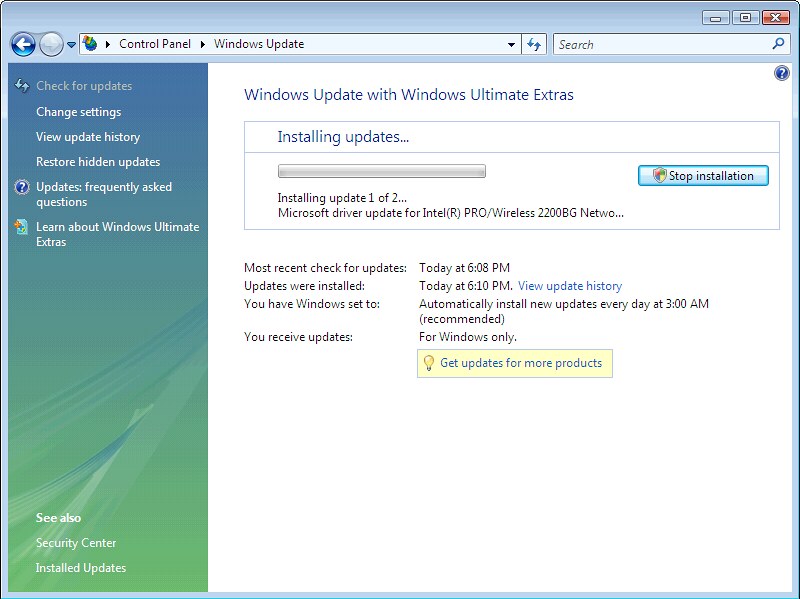The image displays a screen grab of a Windows Update panel within the Control Panel on a computer screen, framed by a blue border. The title panel at the top clearly states "Control Panel - Windows Update," and there is a search bar on the right side of the upper bar. On the left side of the screen, a vertically-oriented menu lists clickable options: "Check for updates" (highlighted in light gray as the current selection), "Change settings," "View update history," "Restore hidden updates," "Updates frequently asked questions," "Learn about Windows Ultimate Extras," "See also: Security Center," and "Installed updates." The background transitions from blue pastel to green pastel toward the bottom.

On the right, in the main white part of the window titled "Windows Update," it shows that updates are in progress under "Windows Ultimate Extras." There is a gray progress bar below, labeled "Installing Update 1 of 2," although it shows no actual progress. To the right is a bright blue "Stop Installation" button. 

Below the progress bar, in black font, is detailed information about the updates: "Most recent check for updates: Today at 6:08 p.m.," and "Updates were installed: Today at 6:10 p.m." A light blue clickable line reads "View Update History." Further details note that "You have Windows set to: Automatically install new updates every day at 3 a.m. (recommended)." 

Underneath in blue font, it states "You receive updates: For Windows only." A yellow box with a light bulb icon indicates, "Get updates for more products," which is also clickable. 

Additionally, the update currently being downloaded is a "Microsoft driver update for Intel® PRO/Wireless 2200BG Network..." (the text cuts off with an ellipsis). The entire interface is designed for managing and tracking Windows system updates.